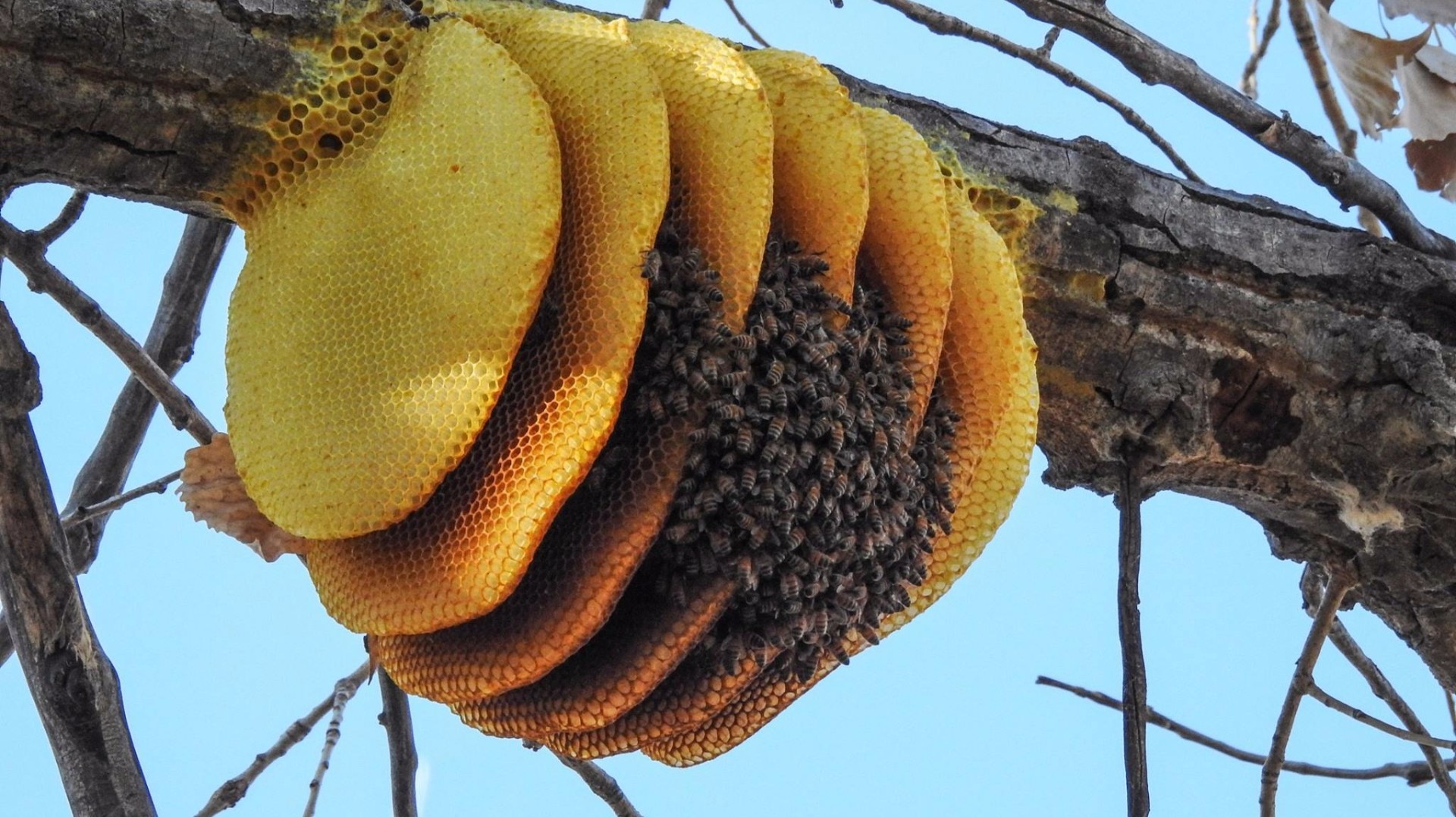This detailed image captures a horizontally hanging beehive attached to a large tree branch with several smaller twigs and limbs protruding from it. The beehive itself features seven distinct layers, each resembling textured discs arranged side-by-side, forming an intricate honeycomb pattern. The color of the hive transitions from a dark brown in the center to lighter shades of yellow towards the edges. The vivid photograph, taken outdoors during a clear day with a bright blue sky, showcases thousands of bees centered within these honeycomb layers. The bees are predominantly black, brown, and yellow, clustering densely within the structure. The encompassing scene also includes the grayish-brown hue of the tree, enhancing the natural contrast against the vibrant hive.